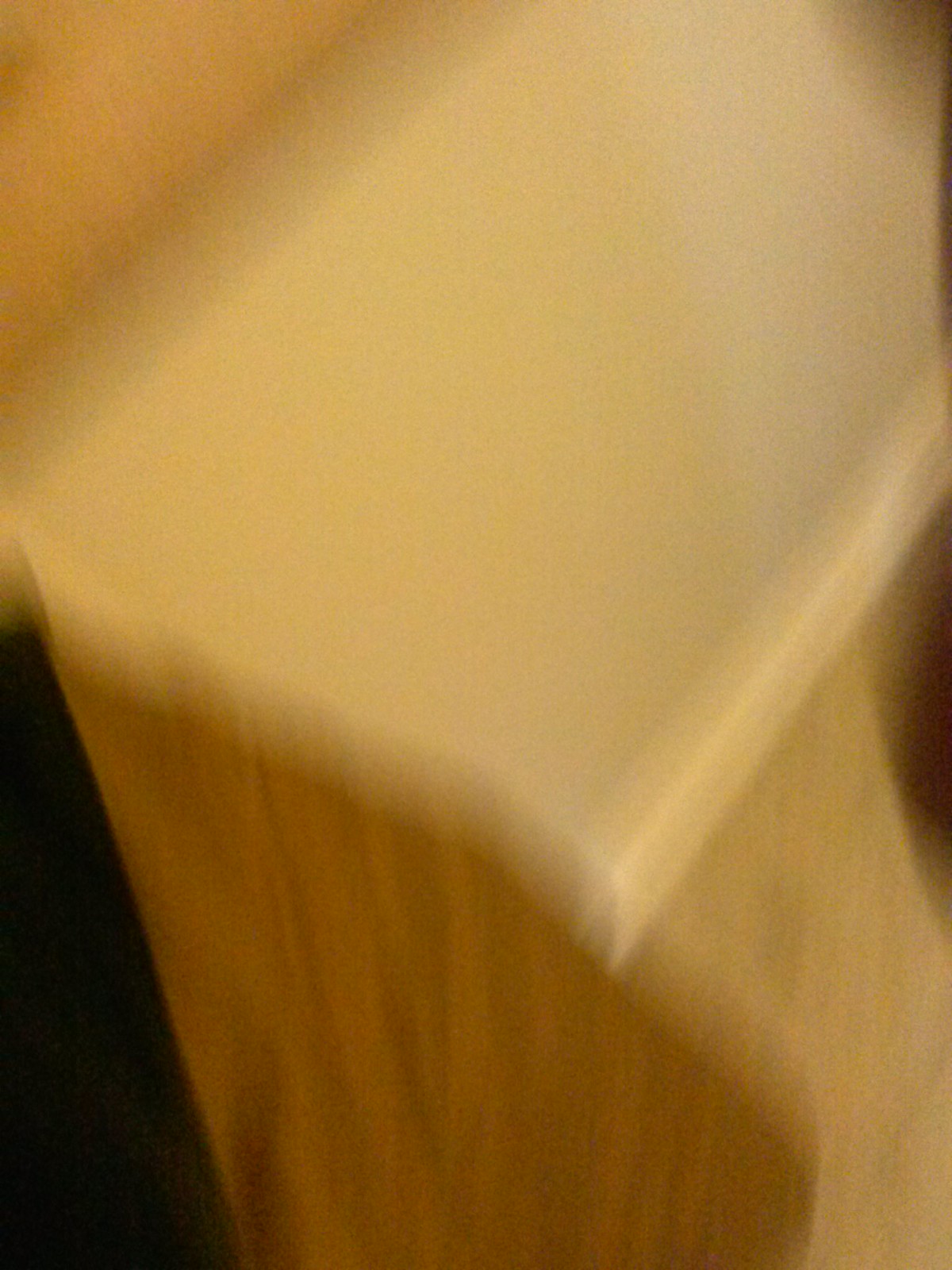This poorly taken photo, blurred and likely shot either in motion or from an extremely close distance, predominantly features shades of beige, dark orange, and black. The central object, seemingly a book or paper due to its rectangular form and curving shape, appears to be bent. In the upper left corner, a portion of what could be the book's spine is visible, with the remaining part partially open. The bottom left corner of the image is notably dark, possibly depicting a sleeve, a body part, or the ground itself. Beneath the lighter rectangular area in the center lies a surface that resembles reddish-brown brick, suggesting it might be the ground or flooring.